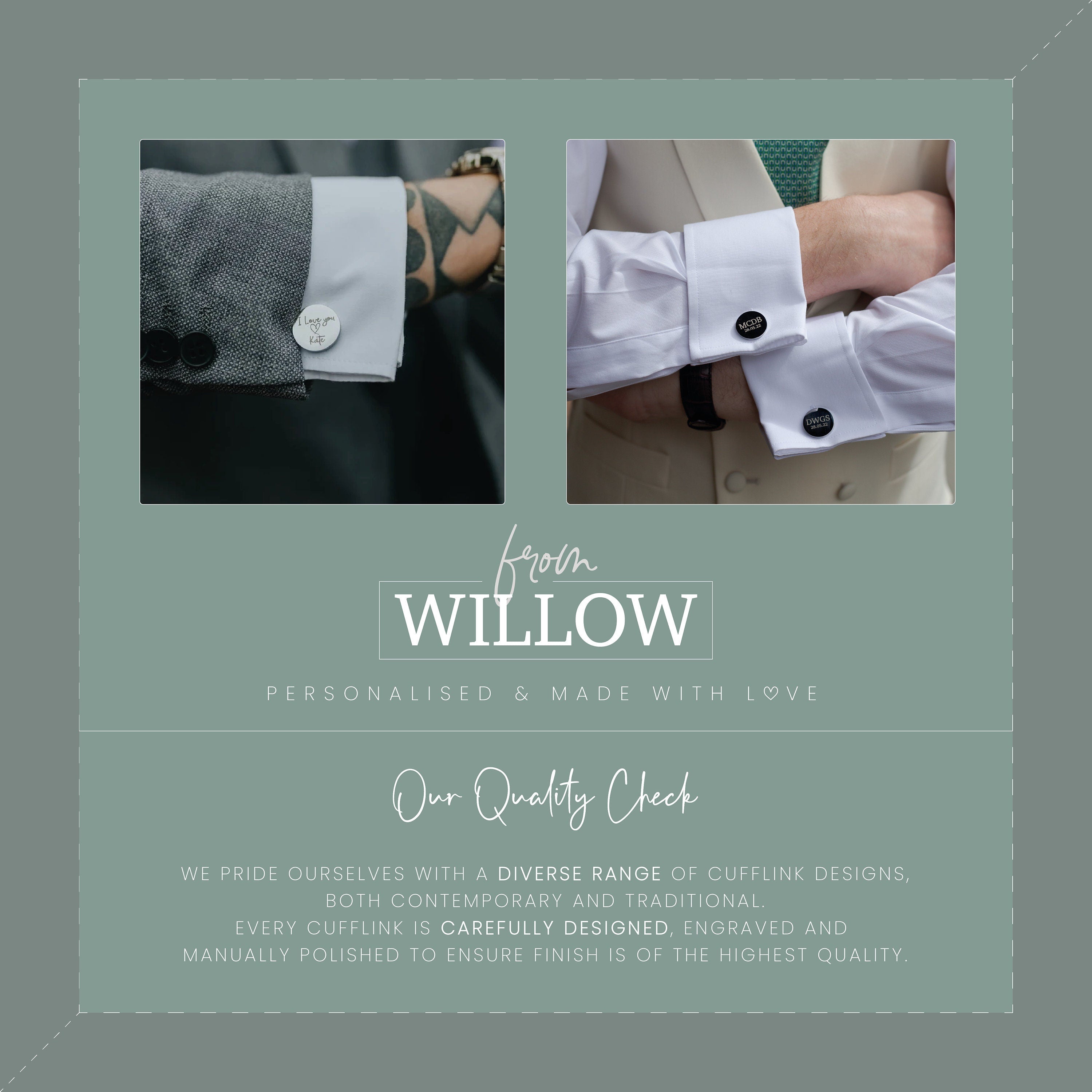This advertisement for men's cufflinks, from the brand From Willow, communicates the message: "Personalized and made with love." The ad highlights their dedication to quality, stating they pride themselves on offering a diverse range of cufflink designs that are both contemporary and traditional. Each cufflink is meticulously designed, engraved, and manually polished to ensure the highest quality finish. 

The ad features two photographs of cufflinks at the top. On the left, there's a man dressed in a gray suit with a golden watch, showcasing a silver cufflink against a muted green background. This man’s forearm is tattooed, adding a unique touch to the stylish presentation. On the right, another man is seen in a beige suit with white sleeves and a black watch, displaying black cufflinks. The background here transitions from a muted green in the center to a darker green on the border, creating a visually appealing contrast that draws attention to the finely detailed cufflink designs.